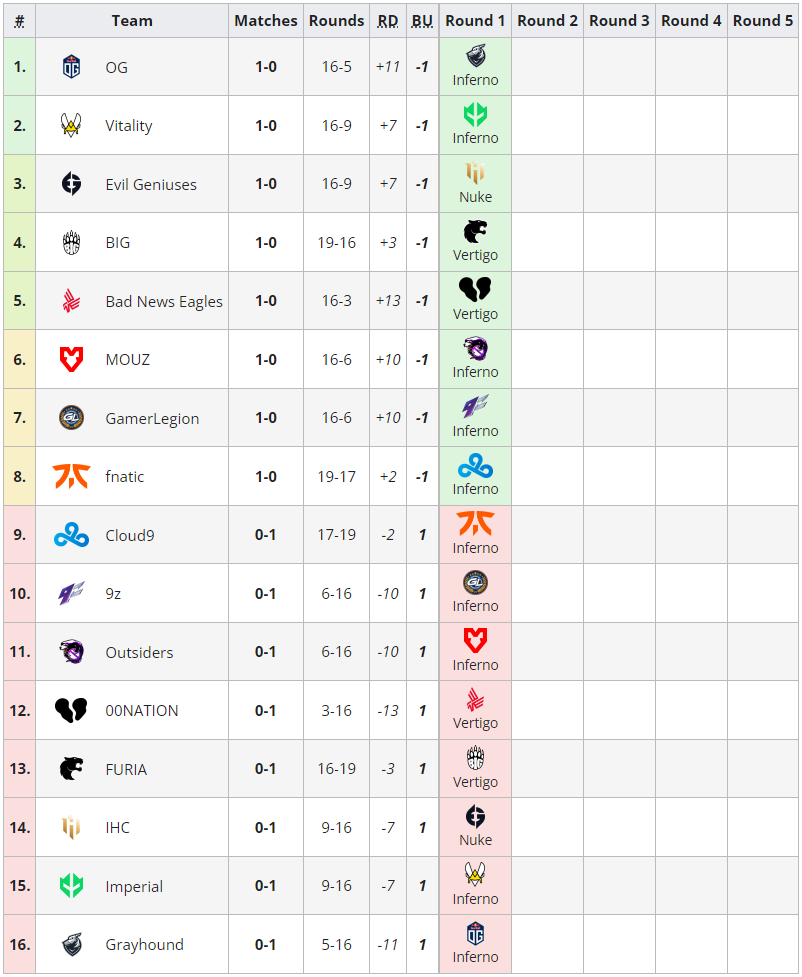The image displays a spreadsheet with a grey background and black font, along with grey headers at the top. The headers include columns for: Number, Team, Matches, Rounds, RD, BU, Round 1, Round 2, Round 3, Round 4, and Round 5.

- Under the "Round 1" column, detailed information is provided for each entry.

1. **OG**:
   - **Number**: 1
   - **Matches**: 1-0
   - **Rounds**: 16-5
   - **RD (Round Difference)**: +11
   - **BU**: -1
   - **Round 1**: Inferno

2. **Vitality**:
   - **Number**: 2
   - **Matches**: 1-0
   - **Rounds**: 16-9
   - **RD (Round Difference)**: +7
   - **BU**: -1
   - **Round 1**: Inferno

3. **Evil Geniuses**:
   - **Number**: 3
   - **Matches**: 1-0
   - **Rounds**: 16-9
   - **RD (Round Difference)**: +7
   - **BU**: -1
   - **Round 1**: Nuke

4. **BIG**:
   - **Number**: 4
   - **Matches**: 1-0
   - **Rounds**: 19-16
   - **RD (Round Difference)**: +3
   - **BU**: -1
   - **Round 1**: Vertigo

Only the "Round 1" column contains data, indicating the map played by each team in their first round.